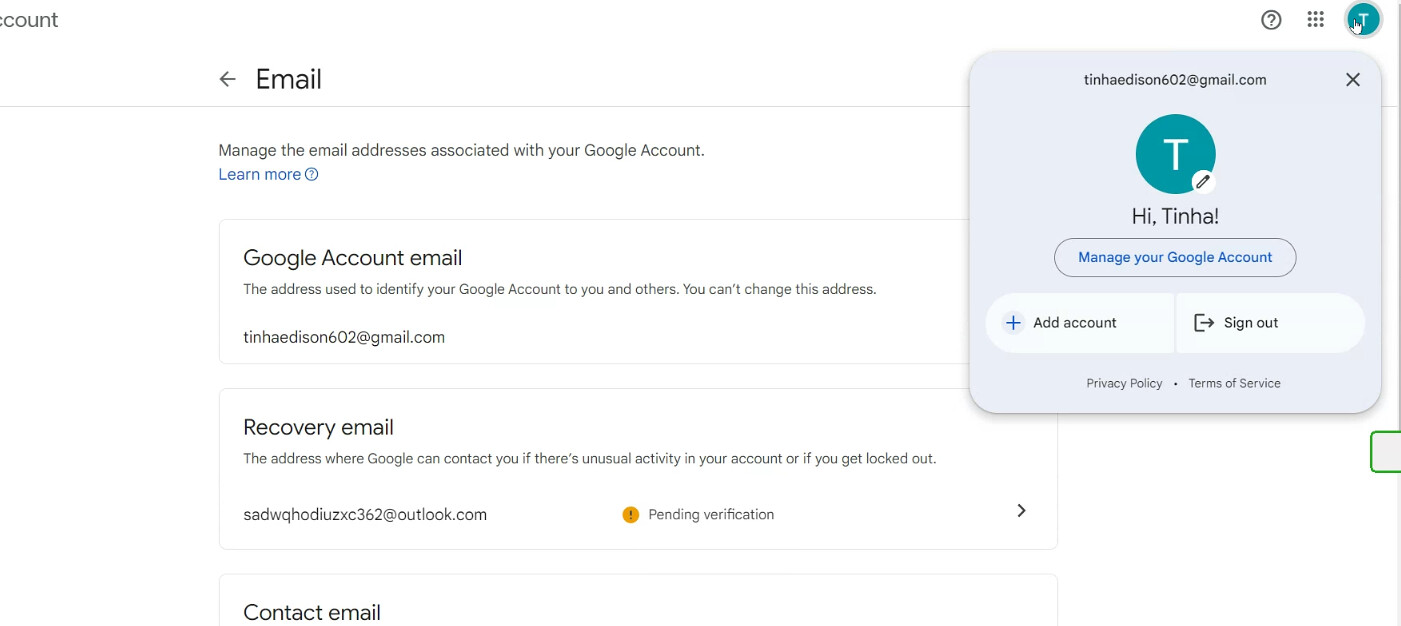Here is a detailed and organized caption based on the provided voice description:

---

The image displays a Google account management page with a predominantly white background. At the top-left corner, the letters "C-O-U-N-T" are visible. About two inches to the right and one inch down, there is a right-pointing arrow followed by the word "email."

Directly below is text in small black letters that reads, "Manage the email address associated with your Google account." Under this, blue text says "Learn more."

There are multiple rectangular sections within the image. The first rectangle contains the header "Google account email" in slightly larger text, followed by the user's email address.

The second rectangle is headed with "Recovery email" in large black letters, followed by additional information and the user's associated recovery email address, which is labeled "Pending verification."

A third rectangle is partially off the bottom of the image and labeled "Contact email" in black text.

In the top-right corner of the image is a small blue circle with a white arrow inside. To the left of this circle, there are three dots arranged in a grid pattern (three across and three down), and further left is a small circle with a black question mark inside.

Below these elements is a light blue square with an "X" in the top-right corner and an email address in the center. Positioned below this is a blue circle with a white letter "T" in the middle. In the bottom-right corner of this blue circle, there is a smaller white circle with a pencil icon inside, indicating an option to edit.

Text in black letters below the blue circle says, "Hi Tina." Underneath this is a blue tab with the text "Manage your Google account." To the left and slightly down from this tab is a white tab with a blue plus sign and the text "Add account" in black. To the right of this tab is another white tab featuring a small C with an arrow pointing to the right, followed by the text "Sign out" in black.

At the bottom of the image, "Privacy Policy" and "Terms of Service" are displayed in black text.